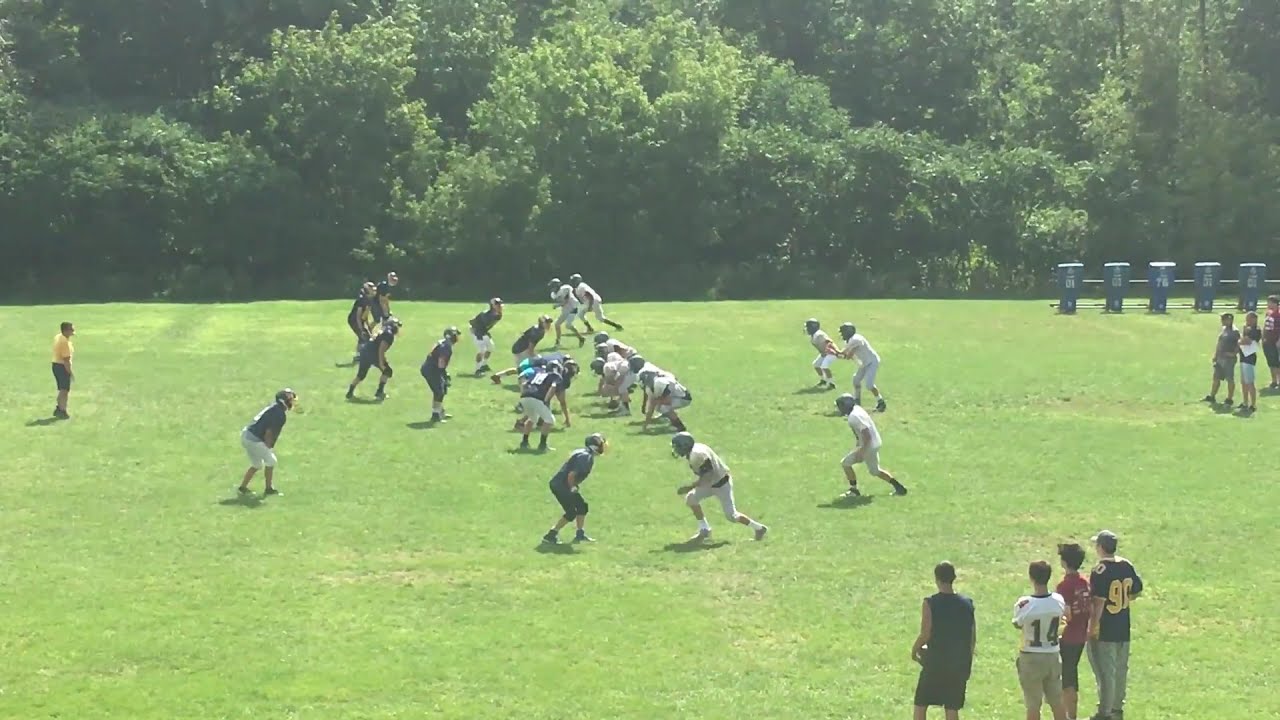The image depicts a lively outdoor football game on a green field surrounded by trees. On the left, players are predominantly dressed in blue shirts paired with either black or white pants, and black helmets. On the right, the opposing team wears white shirts and pants, matched with dark green helmets. Both teams are getting into formation for a play. In the bottom right corner, a few young spectators are wearing jerseys with numbers 14 and 90 or 98, mingling with one person in a plain shirt. A referee in a yellow shirt and black pants is visible on the far-left side. Above the spectators on the right, blue and white football practice equipment can be seen, while in the background, trees frame the entire scene. Standing behind to the right and left, a handful of people observe the game, adding to the bustling atmosphere of this football event.